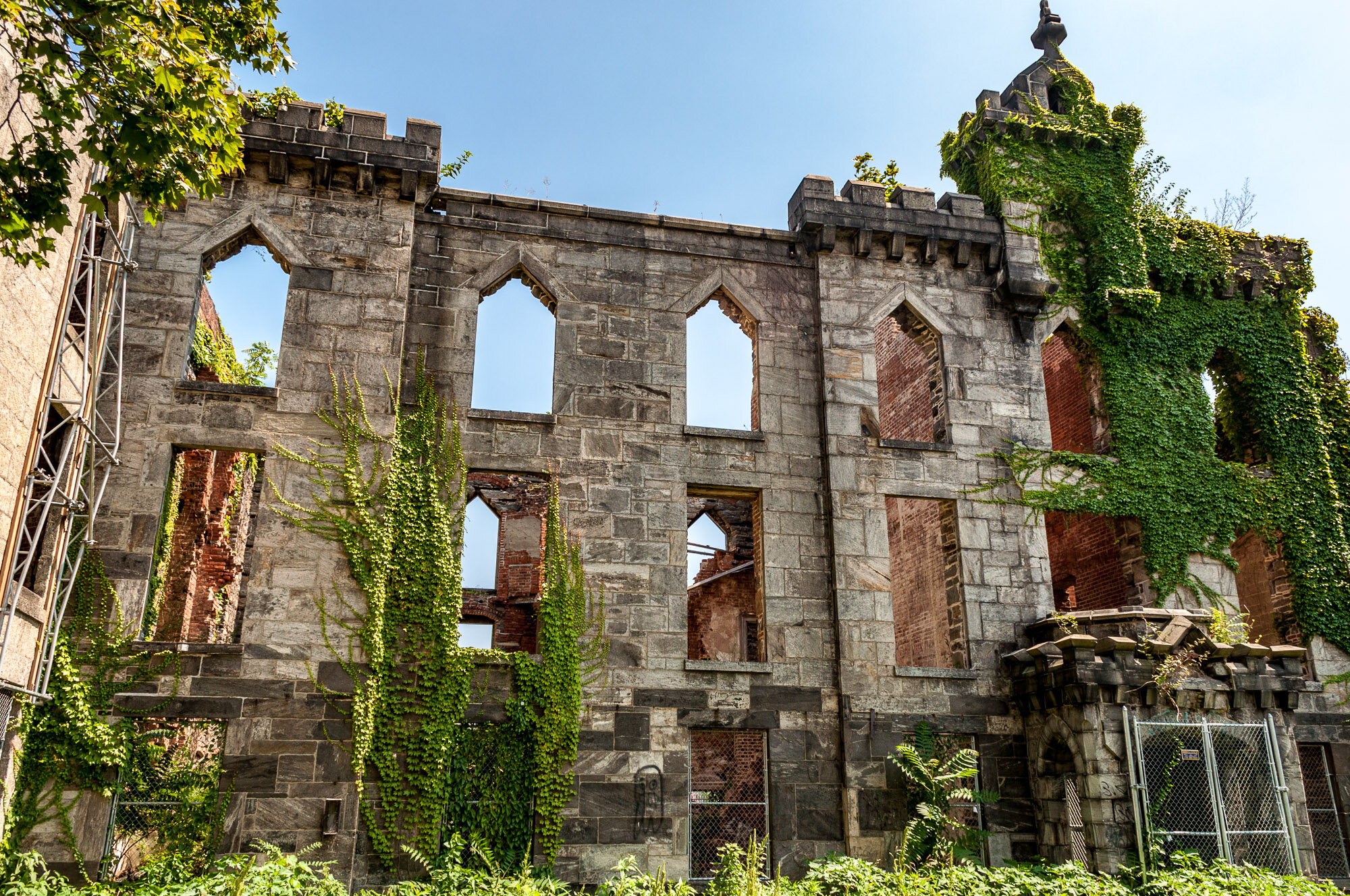This photograph captures the hauntingly beautiful ruins of an old church. The church facade, made of aged gray stone or brick, stands as the most prominent feature, its detailed architecture still apparent despite the absence of a roof and windows. Moss and various climbing plants, including ivy, have overtaken parts of the structure, with foliage cascading from the ground up on both sides. This verdant growth creates a striking contrast against the weathered stone. The facade is punctuated by sky glimpses visible through the empty window frames, with the sky appearing as a light blue gradient that becomes brighter toward the upper right corner. Although the site exudes an inviting aura for exploration, safety measures, such as fencing, have been implemented around the entrances to prevent unauthorized access. The photograph beautifully captures the intertwining of human history and nature’s resilience, making the ruins a captivating, if somber, landmark.